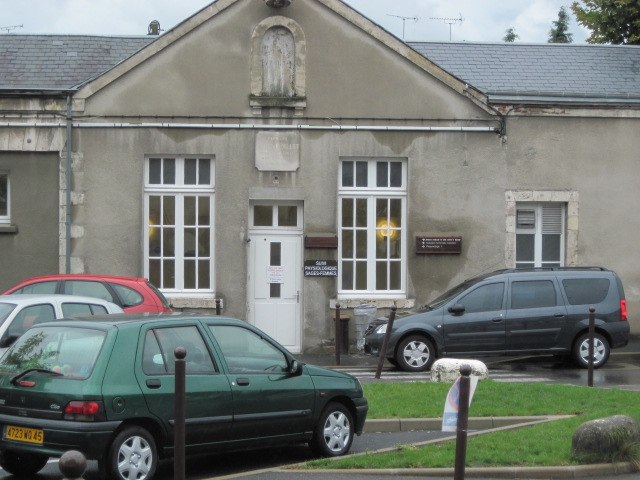The image showcases an outdoor scene featuring a gray cement building with a triangular-shaped shingle roof, possibly an old school. The sky above is gray with scattered white clouds and tree leaves are visible in the top right corner. The building's front facade includes a white door centered between two tall windows, both outlined in white, and another window on the right-hand side. A brown plaque with white lettering is mounted on the wall to the right of the door, and lights are on inside the building, visible through the windows. In front of the building is a roadway and a parking lot where several cars are parked: a gray SUV, a red van, a white car, and a green car. The parking lot is surrounded by posts and patches of grass, and the ground appears wet, indicating a rainy day.